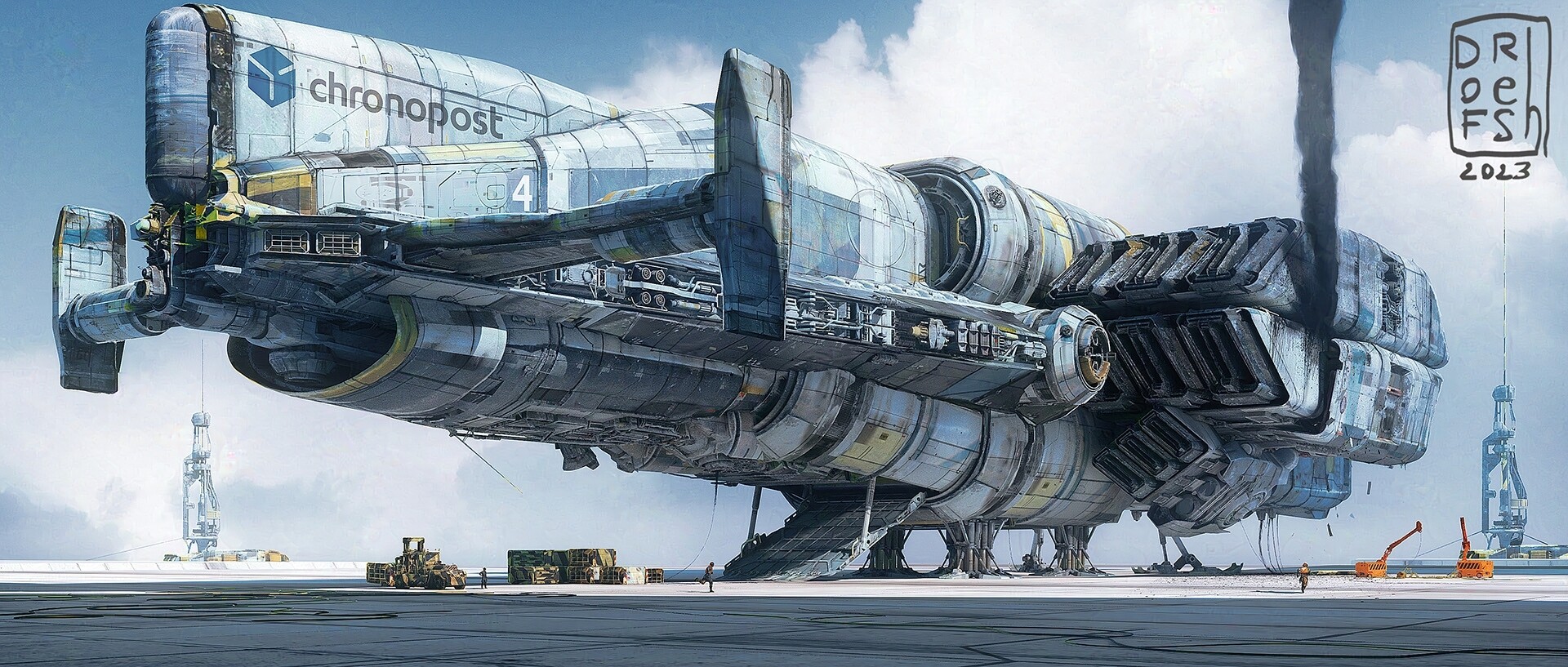The image depicts an artistic rendition of an enormous sci-fi spaceship reminiscent of something from the Star Wars universe, displaying the name "Chronopost" along with a logo and the number "4" on its hull. The vehicle, primarily illustrated in shades of grey, blue, and white, features light blue and yellow accents. It has a tube-like structure with thrusters on the back, and a plume of black smoke is rising skyward from it. The foreground reveals dwarfed military-green trucks and yellow construction equipment beneath the hulking ship, along with small human figures moving nearby. The scene also displays a few orange cranes and two sci-fi-looking skyscrapers in the background, contributing to the futuristic setting. Additionally, in the upper right corner is a stylized mark that appears to read "Dr. D-O-F-R-E-S-H," hinting at an author's signature or a reference.